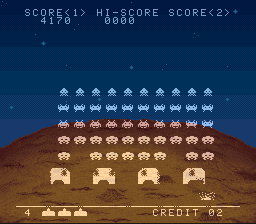The screenshot captures a nostalgic moment from the classic video game, "Space Invaders." The scene is set against a dark blue, star-speckled background, evoking the vastness of outer space. A brown, slightly curved surface at the bottom hints at the ground or a hill, adding depth to the image.

At the top of the screen, the game's UI displays in light blue text: "SCORE" with the number 1 in parentheses beside it, and "HIGH SCORE" with the number 2 in parentheses. The current score is proudly shown as 4,170, while the high score section, disappointingly, remains at 0000, indicating no successful high scores yet.

Midway down the screen, a formation of classic Space Invaders begins their ominous descent. They're lined up in rows, ready to be fought off by the player. At the very bottom, a series of bases or bunkers are positioned as defensive structures, emerging right above a thin horizontal line.

Below this line, the number 4 is stationed on the left, likely indicating the player's remaining lives. Adjacent to this, three small graphical icons represent the bases or guns available to the player, and a notation of "2 CREDITS" is visible, indicating the number of credits inserted into the game.

This evocative screenshot captures the essence of early arcade gaming, where simple graphics and straightforward mechanics combined to create an engaging, timeless challenge.